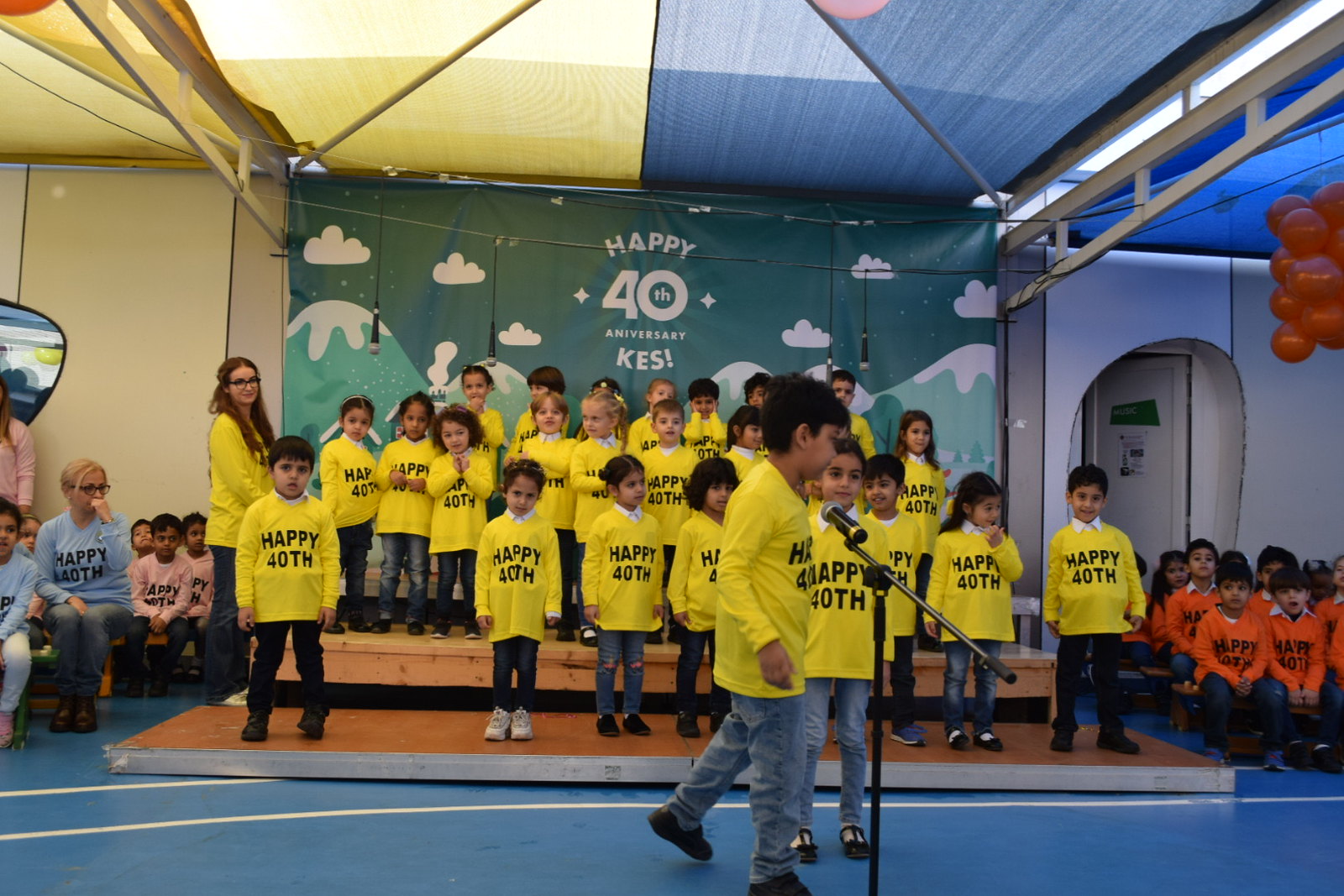This image captures an indoor event, likely a school's 40th anniversary celebration organized by KES. The main focus is a group of young children, all under the age of eight, standing on a stage and bleachers. They are predominantly dressed in yellow long-sleeved shirts with "Happy 40th" printed in black text. Flanking the central group on stage are kids in various other colored shirts: on the left, children wearing pink shirts and a couple in blue; on the right, kids dressed in orange-peach shirts. All the shirts bear the same "Happy 40th" inscription.

A teacher with long, golden-brown hair, also wearing a yellow "Happy 40th" shirt, stands to the side. In the forefront, two children are at a microphone, preparing to address the audience, while the seated kids appear to be around five to seven years old.

The background features a vivid green banner with snow-capped mountains and clouds that reads "Happy 40th Anniversary KES." Adding to the festive atmosphere, a cluster of orange balloons is situated near the upper right corner. The setting is likely a gym, as suggested by the blue floor with white stripes. The main colors in the scene are yellow, green, blue, and orange, with hints of pink, making for a lively and colorful celebration.